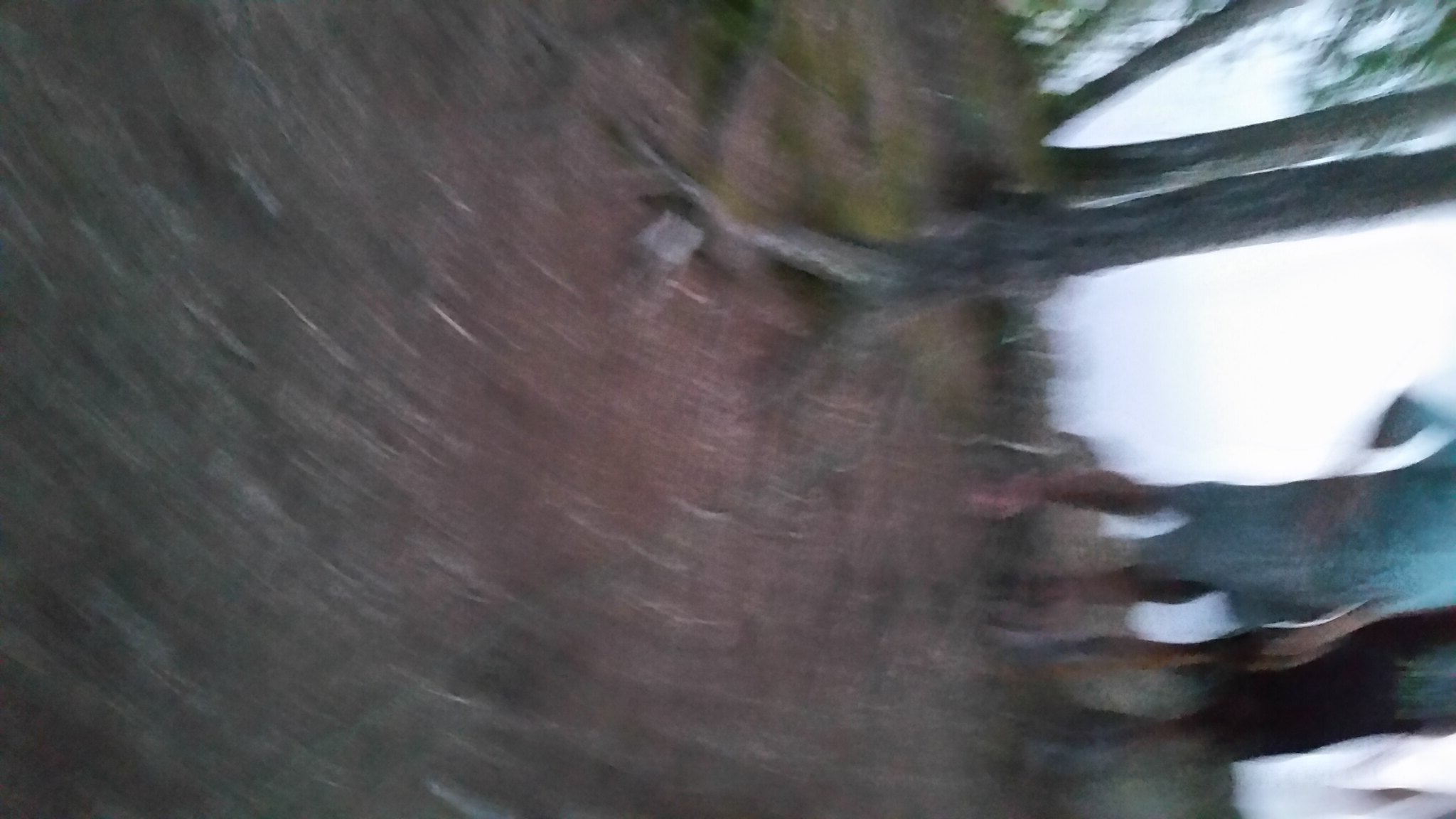This image, captured in extreme blurriness, depicts an outdoor area, potentially a forest or a campground beside a lake. The photograph appears to be tilted 90 degrees, making it difficult to discern specific details. Dominating the center is a swirl of gray, green, brown, and pink hues, creating a hazy, almost abstract appearance. As the blur diminishes toward the edges, several elements become slightly more distinct. Light gray or brown tree trunks stand amidst green leaves, with their roots visible on the ground. The ground itself is a mixture of grass, red and brown dirt, and moss-like patches. Cloudy skies occupy the right-hand side of the image. Toward the top-right (or right side, considering the horizontal flip) stand two people, one donning a black outfit and the other in a light blue ensemble, though exact details remain indistinguishable due to the overall lack of focus.